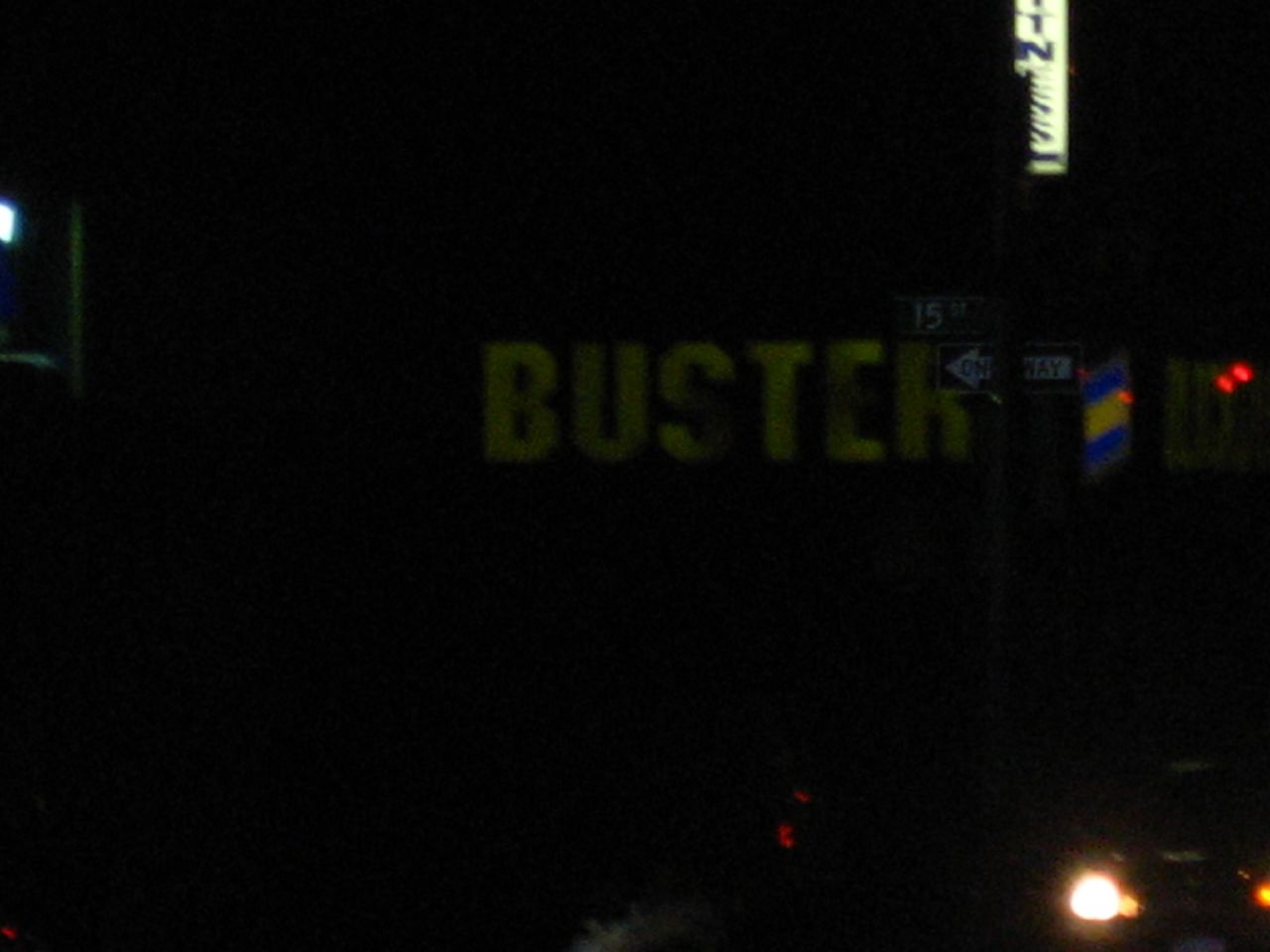In this horizontal image taken outdoors at night, the scene is predominantly pitch black, creating a stark contrast with the scattered lights. The most prominent feature is the word "BUSTER," written in faint white letters across the upper center of the image, set against the dark backdrop. This appears to be on either a building sign or the side of a wall. In the top right corner, there's an illuminated sign with blue letters. Near the middle right-hand side of the picture, a one-way street sign, possibly indicating "15" or "15th Street," is mounted on a pole, with a slight arrow visible. Various lights punctuate the darkness: pairs of small red dots are visible on the right side and bottom middle, a long white spot is at the top right, and a bright white car light is conspicuous in the lower right-hand corner. Additionally, a red light, featuring blue and gold stripes, adds a splash of color to the right side of the image.